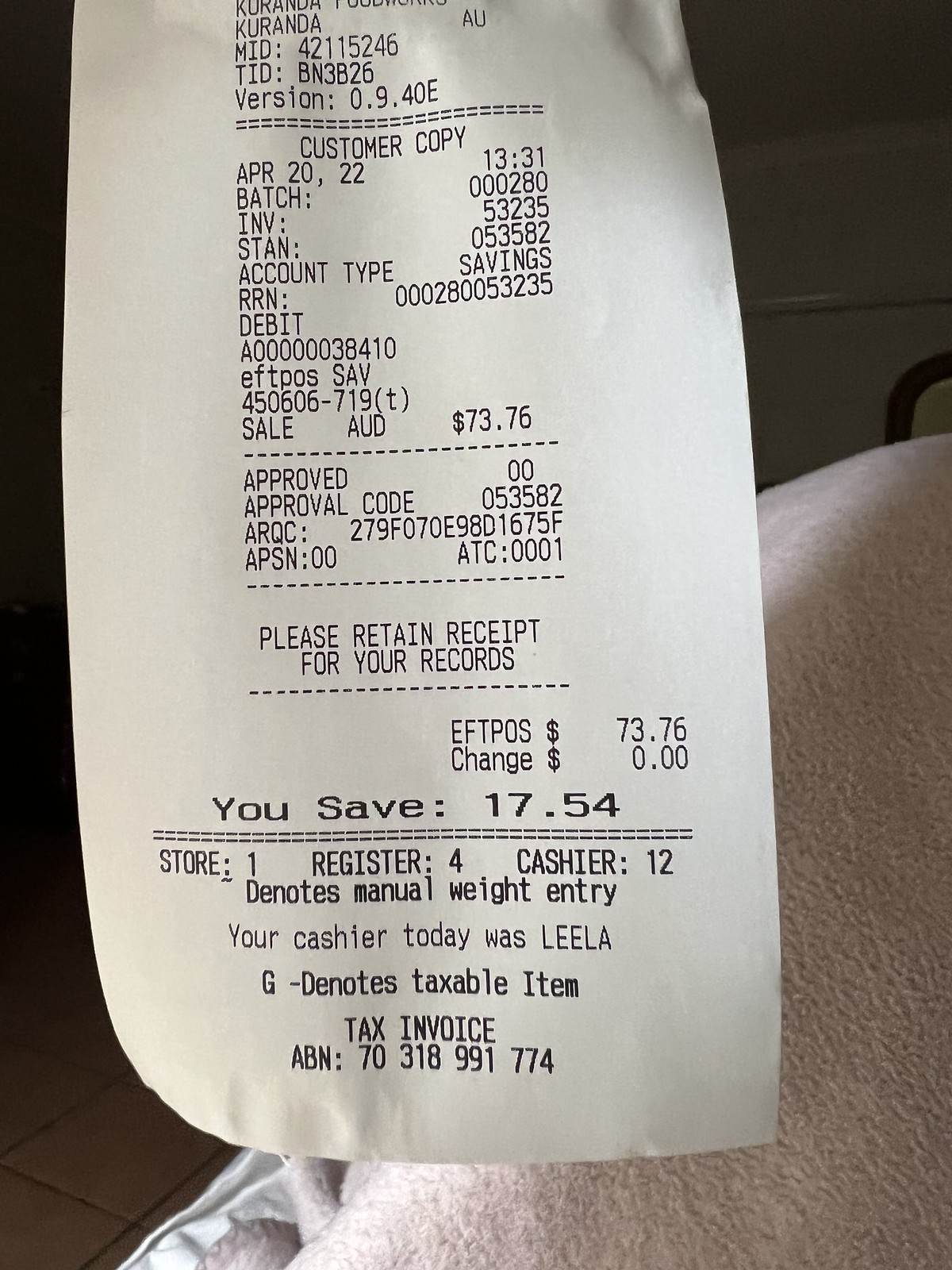This image captures the bottom half of a receipt. The receipt details are as follows: 

Karanda MID: 42115246  
TID: BN 3B26  
Version: 0.9.4 DE  
Customer Copy  

Date: April 28, 2022  
Time: 13:31 PM  

Batch: 000280  
Invoice: 53235  
Stan: 053582  
Account Type: Savings  
RRN: 000280053235  

Transaction Details:  
Debit: $73.76  
Additional Charge: $17.54